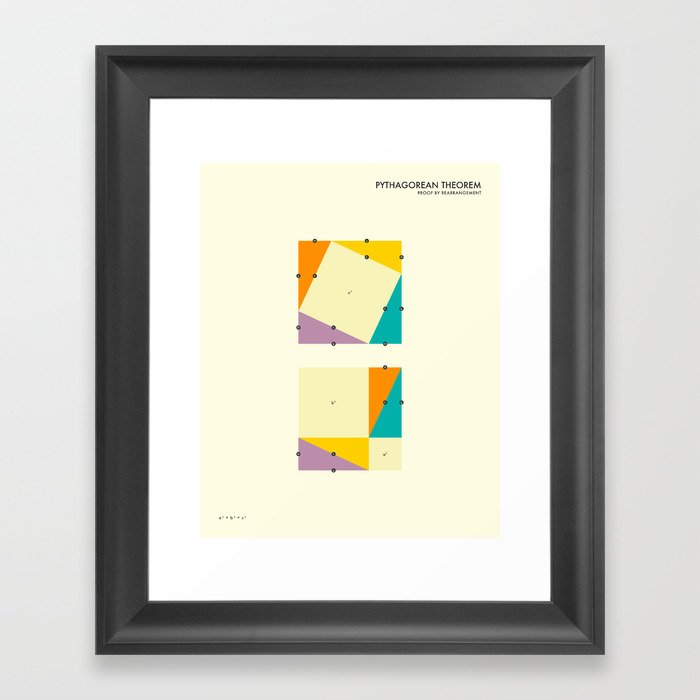This photograph features a wall-hanging picture frame of the Pythagorean theorem. The frame, which is matte black and appears to be wooden, contains a white matting with a vertical rectangle of light yellow in the center. At the top of this rectangle, the text "Pythagorean Theorem" is clearly visible. Below the title, there are two geometric illustrations. The upper illustration is a large skewed square surrounded by four rectangles, distinctly highlighted by colorful triangles: a small orange triangle on the left, a yellow triangle on the top right, a teal triangle on the bottom right, and a purple triangle on the bottom left. The lower illustration, similar in appearance, also features a colorful composition of triangles and squares, visually explaining the Pythagorean theorem with a harmonious palette of light yellow, yellow, orange, purple, and turquoise. The entirety of the artwork effectively blends mathematical precision with artistic design.